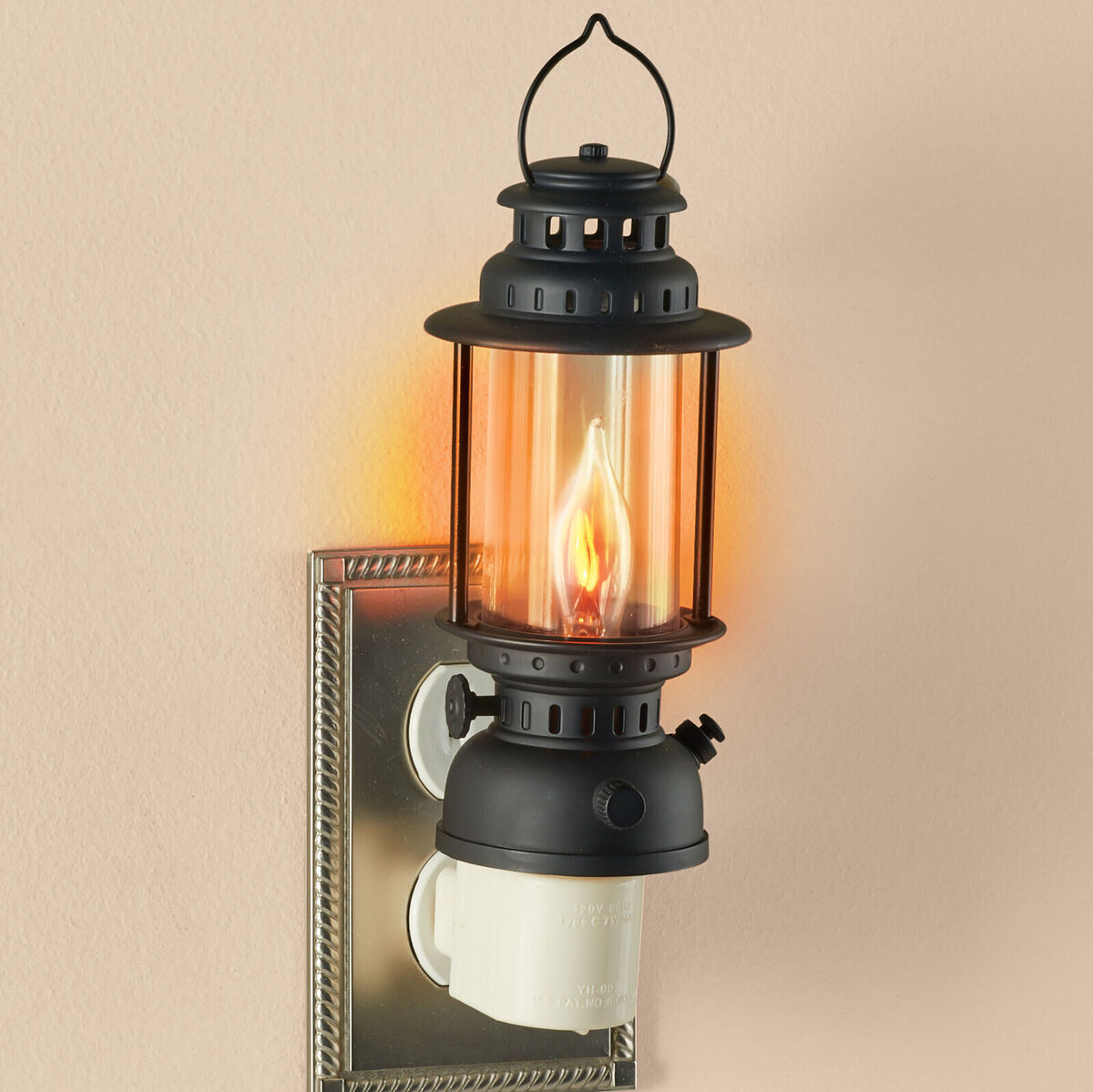This photograph showcases a black, metallic-looking nightlight designed to resemble a miniature lantern, plugged into the bottom socket of a white outlet inset within an ornamental, silver-colored faceplate. The lantern nightlight features a small, flame-like orange bulb encased in a glass tube, and its black metal frame mimics the structure of a full-sized lantern complete with a rounded handle on top. The outlet is mounted on a smooth, cream-colored wall, adding a warm ambiance to the scene.